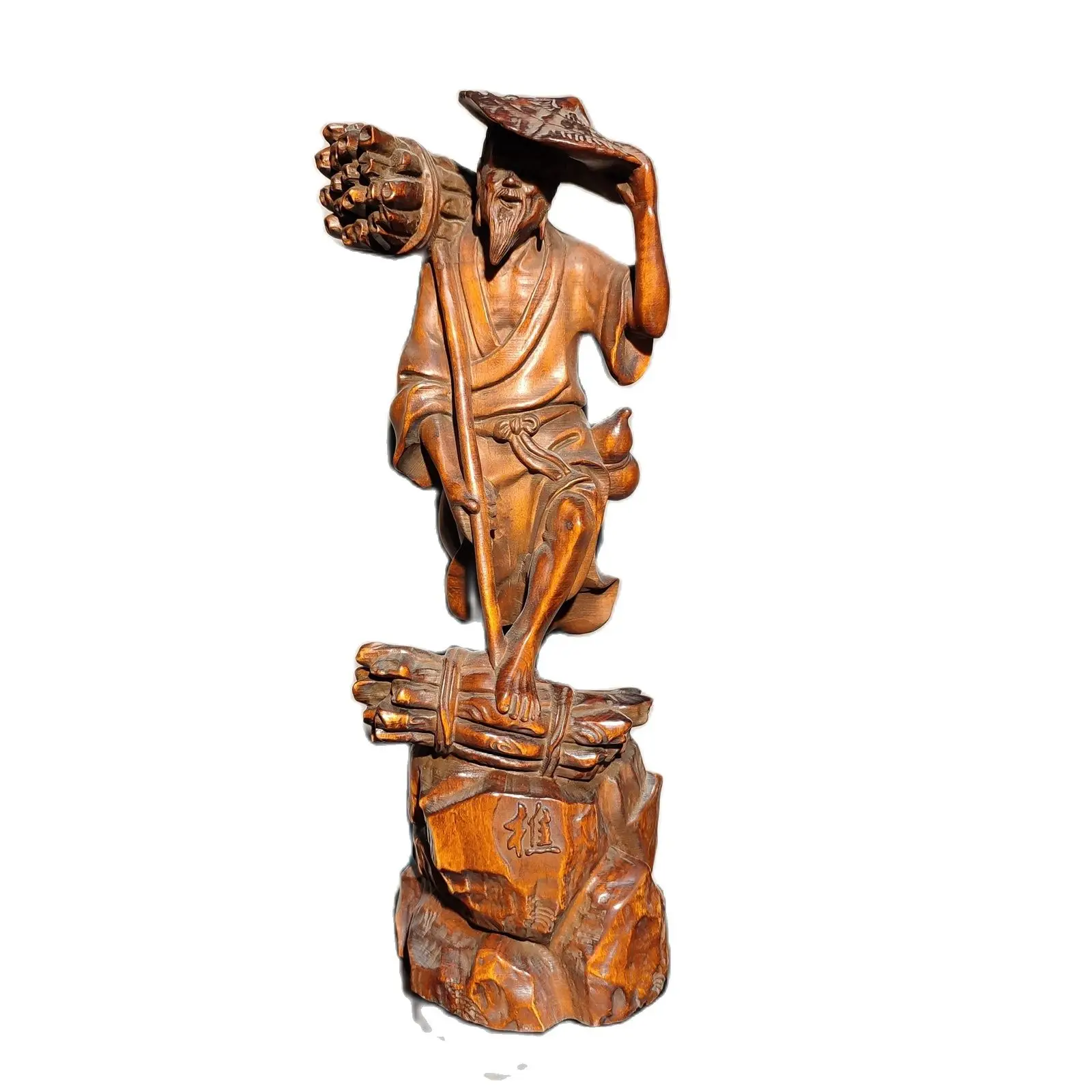The image showcases a detailed wooden sculpture of an elderly Asian man, characterized by a long, pointed beard and a traditional wide-brimmed, pointy hat commonly associated with agricultural work in Asian culture. The man stands on a pile of rocks inscribed with Chinese or Japanese symbols. His right arm extends downward holding a staff or cane, while over his right shoulder rests a bound bundle of firewood. His left hand steadies his hat, casting a shadow over his face, which is largely obscured. He wears a loosely tied robe that reveals parts of his arms and legs. His left foot is placed on another rolled-up bundle of wood below him. The entire scene is carved from wood, with a light golden-brown hue that highlights the grain and textural details of the material. The background is clean and white, ensuring the focus remains on the intricate craftsmanship of the statue.